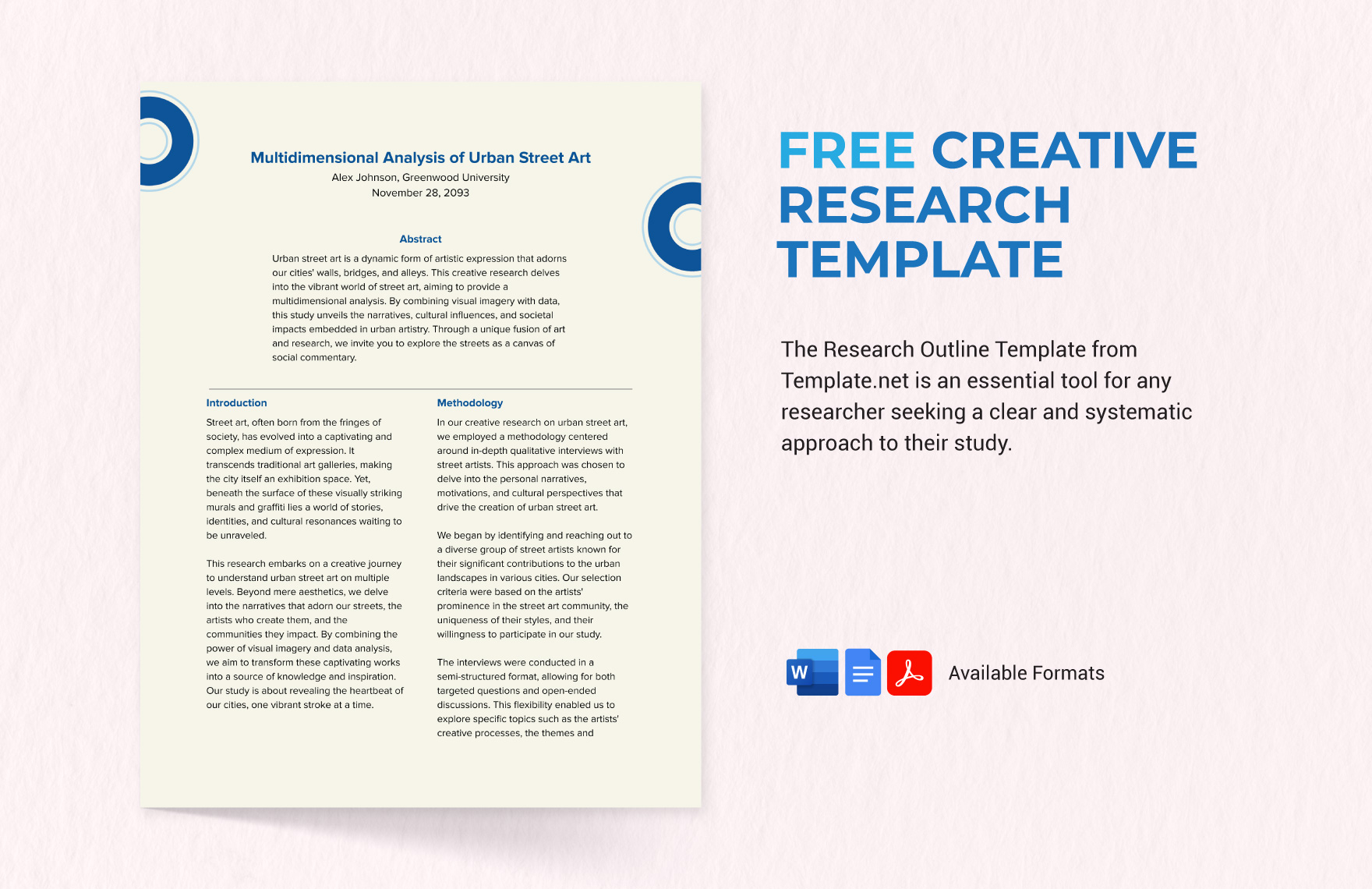The image is an advertisement for a free creative research template, prominently featuring the phrase "Free Creative Research Template" in blue text on the right side. The word "Free" appears in a lighter blue than the rest of the phrase. Below this heading, a paragraph in black font emphasizes that the Research Outline Template from template.net is an essential tool for researchers seeking a clear and systematic approach to their studies. 

A few spaces below the paragraph, icons for Microsoft Word, Google Docs, and Adobe PDF are displayed, accompanied by the text "Available Formats." The background of the image has a textured paper-like appearance, giving it an authentic, tactile look. 

The template itself is shown on a tint of very pale green paper, bordered by circular designs on either side. The header on the template reads "Multidimensional Analysis of Urban Street Art" in blue font. The sample page includes sections for the Abstract, Introduction, and Methodology, providing a glimpse into the detailed structure that researchers can expect from the template.